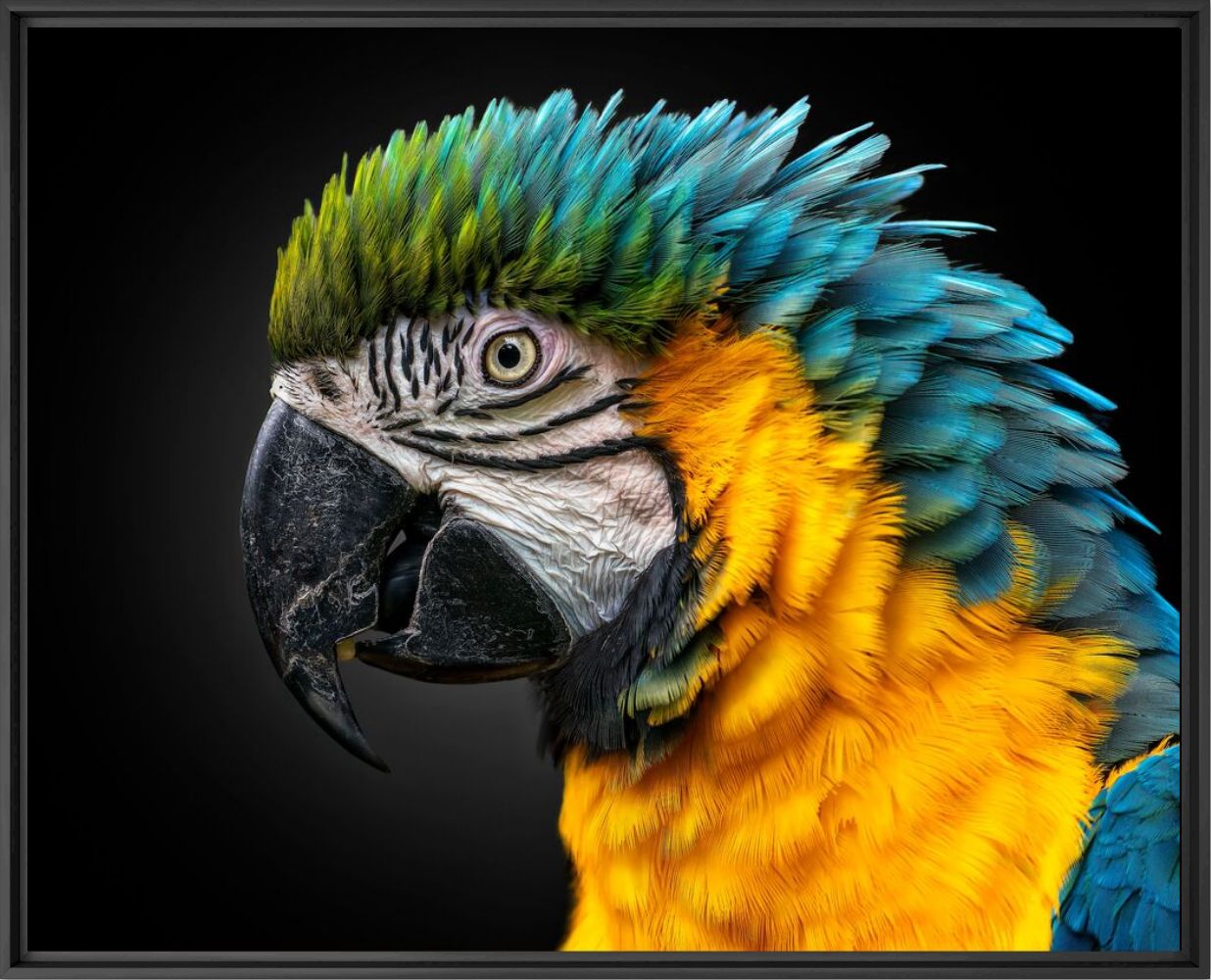This image showcases a vibrant, close-up portrait of a parrot set against a stark black background, causing the bird's stunning colors to truly stand out. The parrot's head features a gradient of feathers that transition from green at the beak, into teal and turquoise, and finally into a darker blue towards the shoulders and wings. The bird's face is predominantly white, accentuated with intricate black lines around its pale, greenish-yellow eye. The sharp, overlapping beak is black and adds to the bird's intense, stoic expression. Its breast and near its ears exhibit a bright, vivid orange-yellow color, giving a striking contrast. This detailed and dynamic portrayal beautifully captures the parrot's posture and the texture of its soft, abundant feathers.